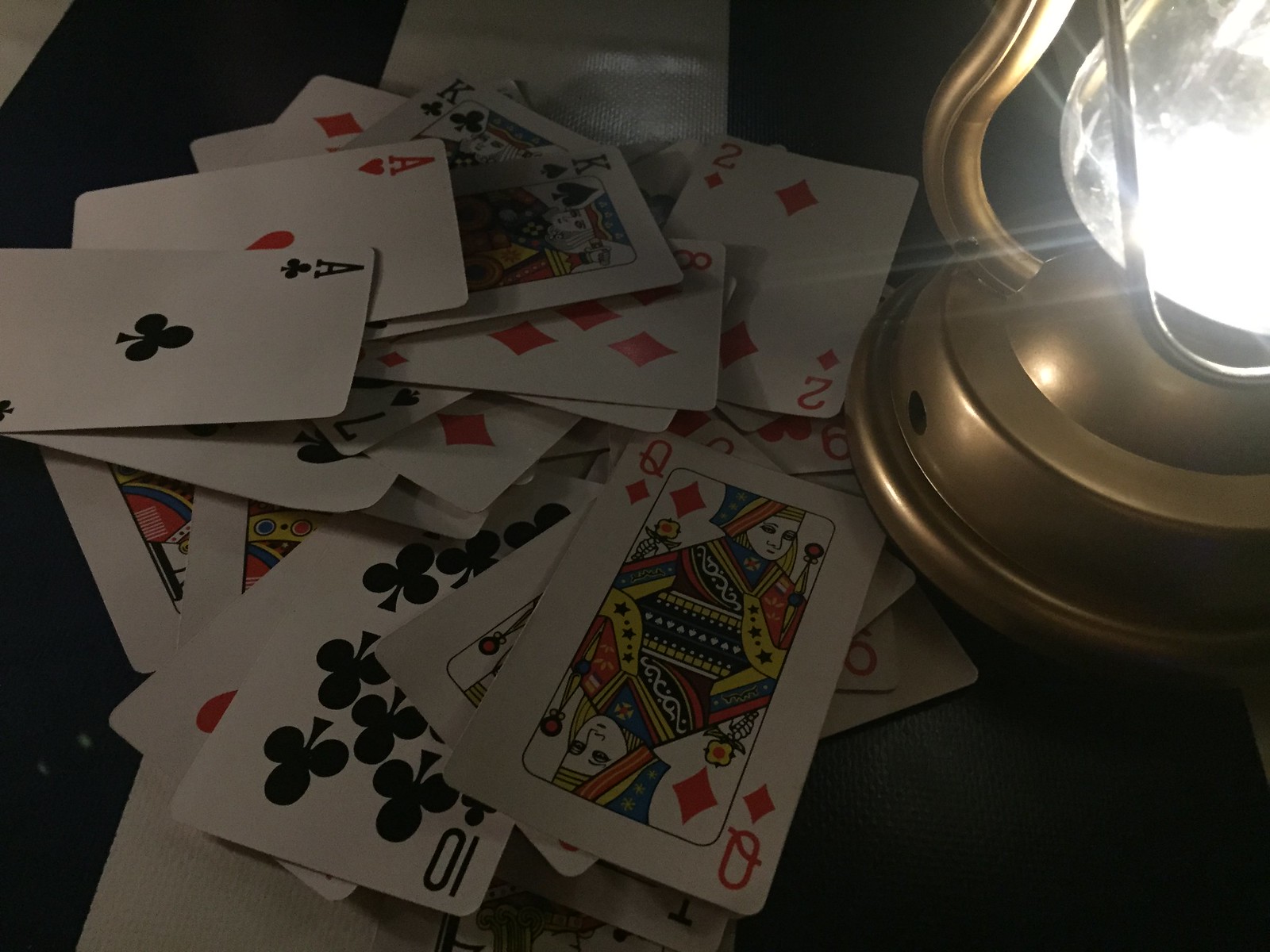The image features a composition with diverse elements and contrasting tones. In the upper left-hand corner, there is a small white triangle against a predominantly black background. Moving horizontally to the right, the black area continues before transitioning abruptly into an image of a gold lamp. The lamp resembles the type often used for camping trips, complete with a silver handle that hangs down. The lamp's center is notably bright, creating a glowing focal point in the image.

Below the lamp, the lower right-hand side of the image displays a dark green color that gradually fades into black towards the right. The lower left section of the image remains consistently black. Scattered across this lower portion are several playing cards, jumbled together face-up. The identifiable cards include an ace of clubs, an ace of hearts, a king of clubs, a king of spades, an eight of diamonds, a two of diamonds, a queen of diamonds, and a ten of clubs.

The white triangle from the top corner is echoed by a small patch of white beneath the cards, nestled between the dark tones on the right and left ends of the image. This small white section adds a subtle balance to the image's contrasting dark elements.